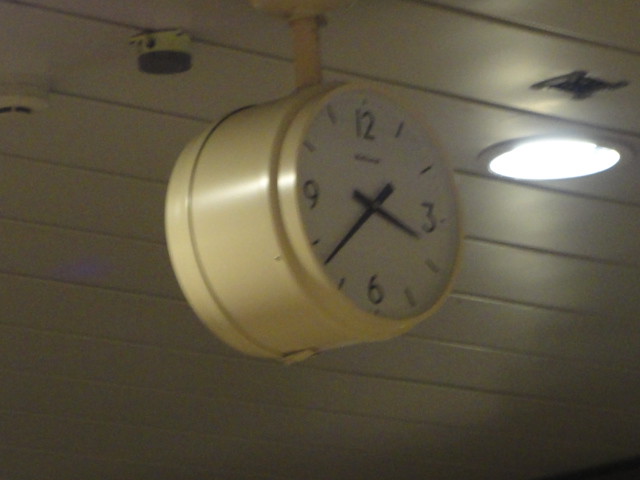This photograph captures a wide clock, possibly designed with dual faces— one visible and the other potentially on the opposite side, connected by a thick band of metal encircling its center. Each face is circular and framed by a light yellow metallic ring. The clock face is white, displaying prominent black numbers at 12, 3, 6, and 9 o'clock positions, with simple black slashes marking the other hours. The time is conveyed by two black hands, one short and one long.

The clock is mounted against a wall painted in a light tan or white hue, contributing to the bright and airy atmosphere of the room. To the right, a ceiling-embedded light fixture adds additional illumination to the setting.